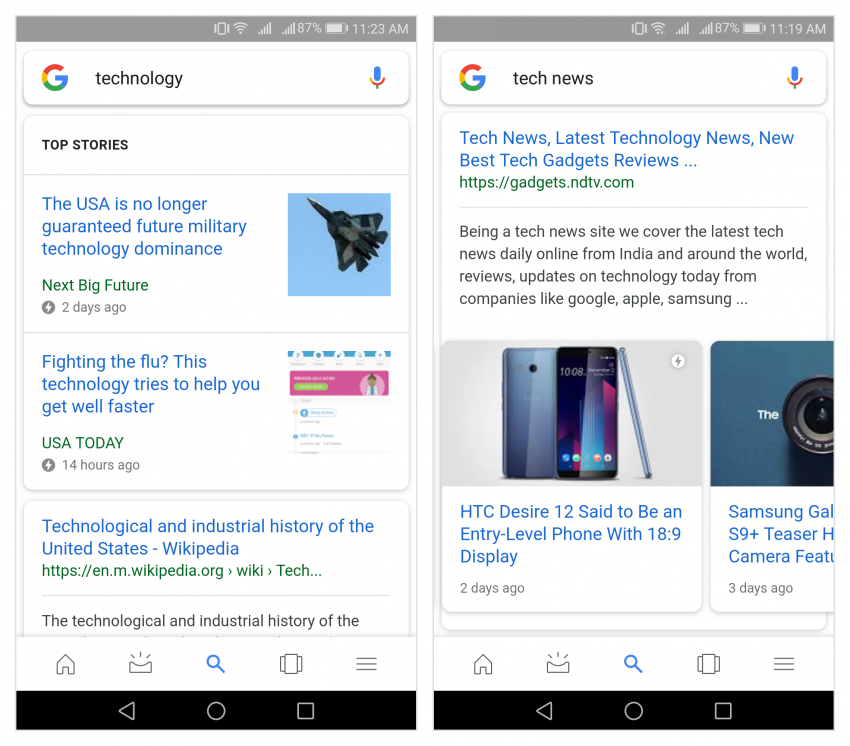This image is a screenshot featuring two side-by-side search results from Google News, captured on a smartphone. Each screenshot displays search results for different queries related to technology. 

On the left, the search query is "technology," and the screen shows a battery level of 87% with the time stamp 11:23 AM. The top stories include:
1. "The US is No Longer Guaranteed Future Military Technology Dominance" by Next Big Future.
2. "Fighting the flu: This Technology Tries to Help You Get Well Faster" by USA Today.
3. "Technological and Industrial History of the United States" by Wikipedia.

On the right, the search query is "tech news," with the screen also showing a battery level of 87%, but with an earlier time stamp of 11:19 AM. The top stories here are:
1. A heading that reads "Tech News: Latest Technology News, New Best Tech Gadget Reviews" leading to a website link at gadgets.ndtv.com.
2. "HTC Desire 12 Said to be an Entry Level Phone with 18:9 Display."
3. The last story, partially cut off, is about the "Samsung Galaxy S9+ Teaser," mentioning a camera feature.

The image showcases how Google News curates and displays news articles based on different search terms and highlights the difference in content between the searches for "technology" and "tech news."